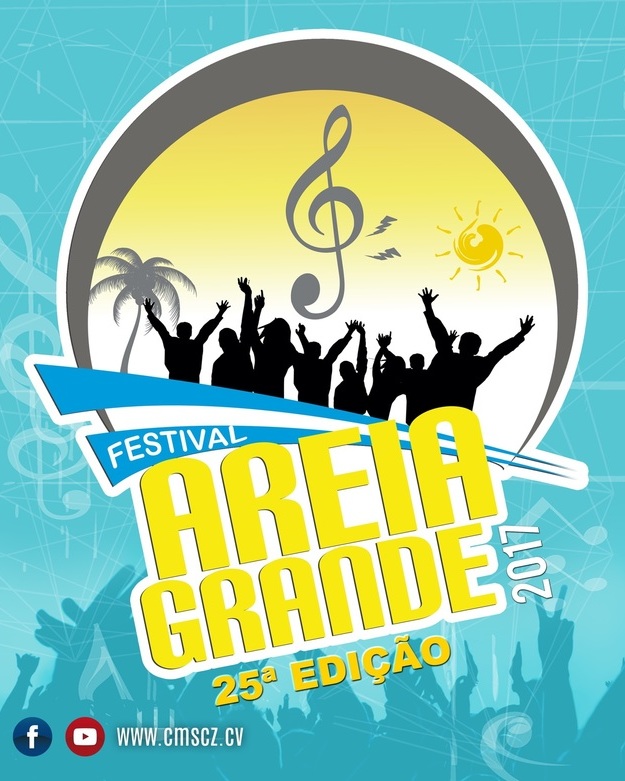The image is a vertical promotional poster for the Aria Grande Festival 2017, set against a seafoam, greenish-blue background. Central to the image is a three-quarters circle featuring a light yellowish background with a gray border. Inside the circle, a musical note is prominently displayed, accompanied by a gray palm tree and a yellow sun on the right. Below these, the silhouettes of approximately eight people can be seen, their arms raised in celebration.

At the bottom of this circle, two blue stripes sandwich a white stripe, with the word "Festival" written in blue on the white stripe. Beneath this, in large yellow letters are "A-R-E-I-A" and "G-R-A-N-D-E" set against a white backdrop, with "2017" placed vertically to the right of "Grande." Below, the number "25" is followed by "EDICAO" in yellow letters, indicating the festival edition. The bottom left corner includes a Facebook icon with a white 'F' inside a blue circle, and a YouTube icon, which is a red circle with a white play button. The URL "www.cmscz.cv" is also displayed.

Throughout the greenish-blue background, various images such as musical notes and additional silhouettes of people with arms raised add a lively ambiance, reinforcing the festival's vibrant, musical theme.